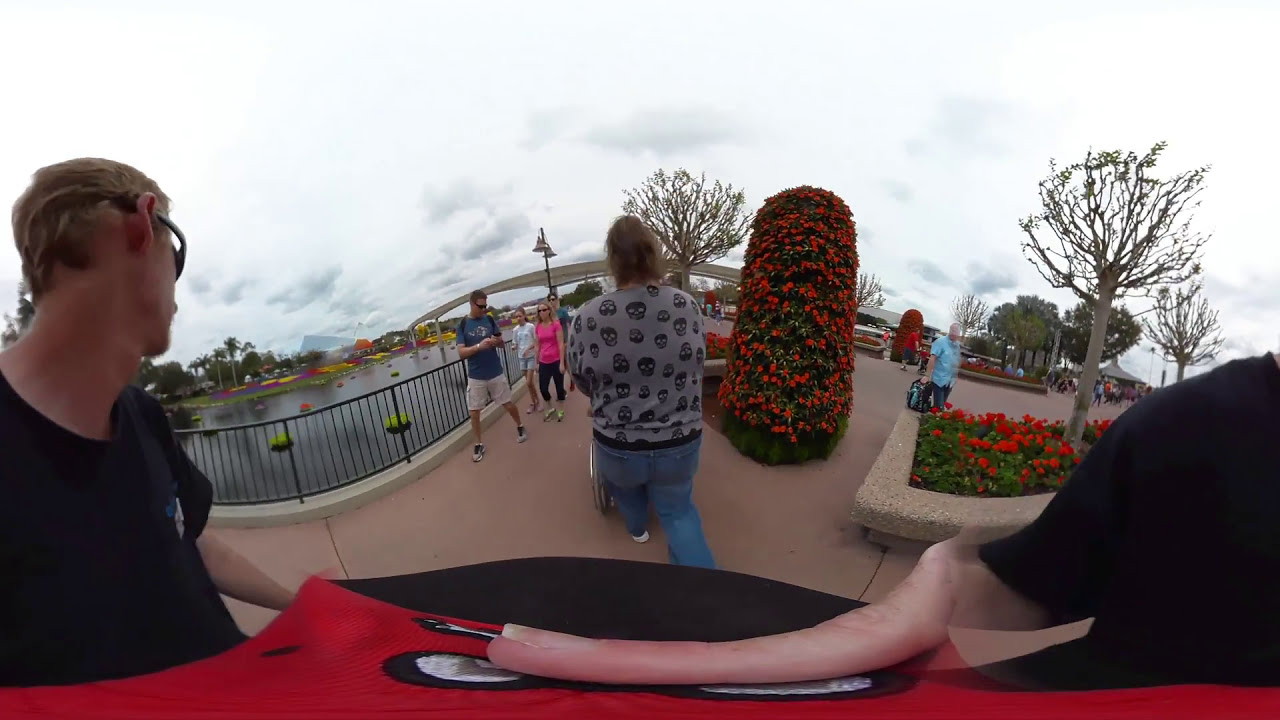The image captures a dynamic and somewhat distorted outdoor scene, presumably in a park or theme park, brimming with various elements and activities. A black metal fence, seamlessly welded into concrete, runs along the border, overlooking a water body adorned with aquatic plants and framed by palm trees. A gray, mostly cloudy sky forms the backdrop, punctuated by patches of gray clouds. 

In the foreground, multiple people navigate the area. To the left, a Caucasian male with short blonde hair, donning a black shirt and sunglasses, appears twice due to the warped nature of the 360° camera, revealing parts of his body in a distorted manner. Nearby, a woman in a gray shirt with black skulls and blue jeans walks forward, pushing either a wheelchair or a stroller on a light brown cement floor.

Central to the image, a man in a blue shirt, cargo shorts, backpack, and sunglasses strides along. Amidst them, a table covered with a red cloth hosts two seated individuals, though part of the scene appears distorted, including a stretched hand.

Red flowers bloom abundantly in a shrub on the right, complemented by colorful yellows and purples elsewhere. A gray monorail track arches overhead in the distance, connecting the vibrant and bustling environment. On both sides of the scene, trees dot the landscape, contributing to the lush surroundings and further enhancing the lively atmosphere.